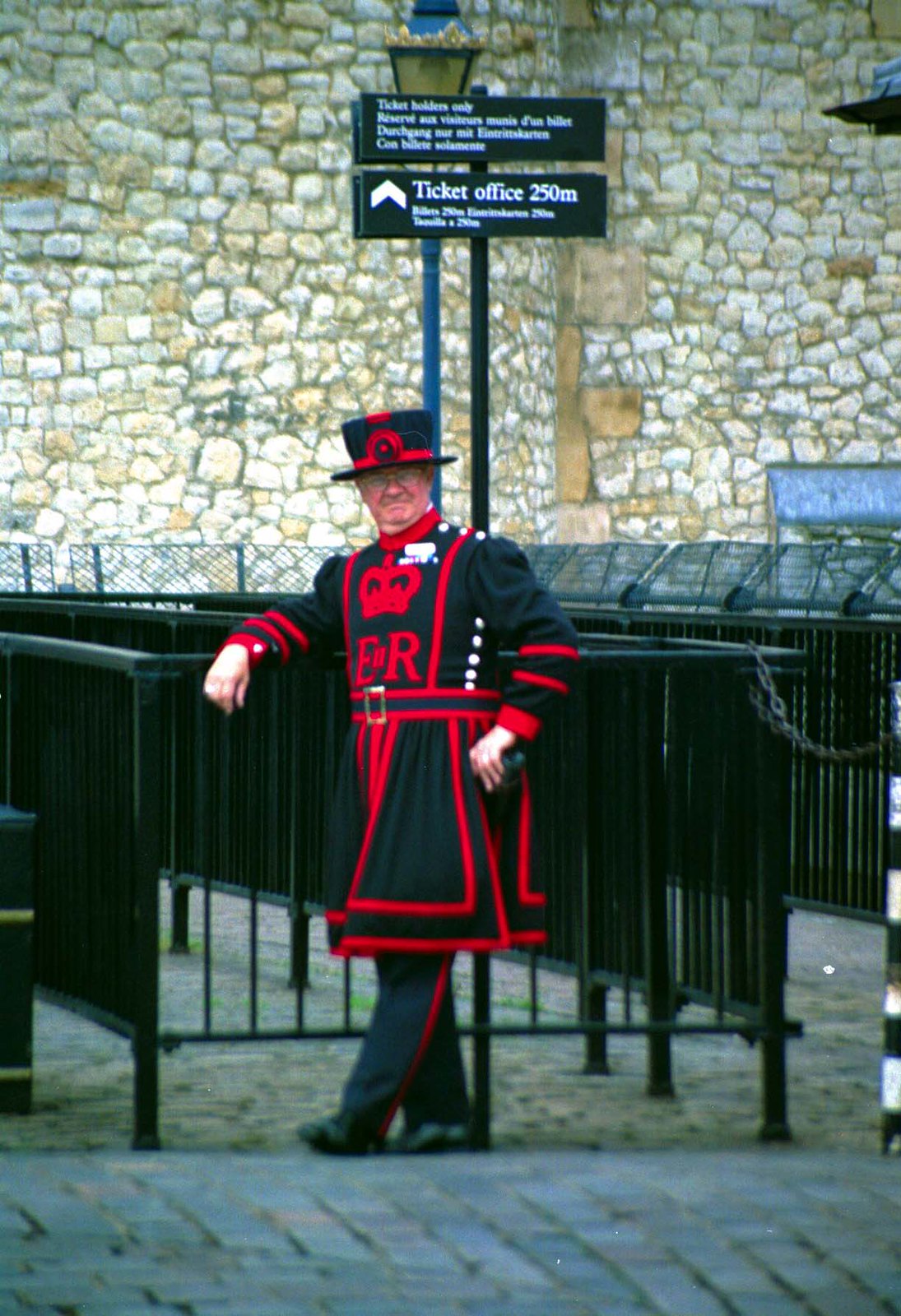The photograph captures a man dressed as a British jester or historical figure, standing in the center of the image. He is wearing an ornate black and red costume, including a long coat with intricate red details, black pants with a red stripe, and black shoes. His attire features a prominent red crown emblem on the front, along with the letters "E" and "R" beneath it. He completes his look with a black and red top hat adorned with decorative elements. The man is leaning against a chest-high black metal fence which seems to be part of an entrance gate, possibly to a museum or historical site. Behind him, a massive stone wall stretches upwards to the top of the image, enhancing the old-world atmosphere. The background also includes a blue light post and black signage with white lettering, with one specified sign indicating a 'Ticket Office 250 meters' away. He acknowledges the camera with a smile, adding a sense of candidness to the historical setting. The foreground features a pathway or sidewalk crafted from stone bricks, contributing to the overall rustic ambiance.